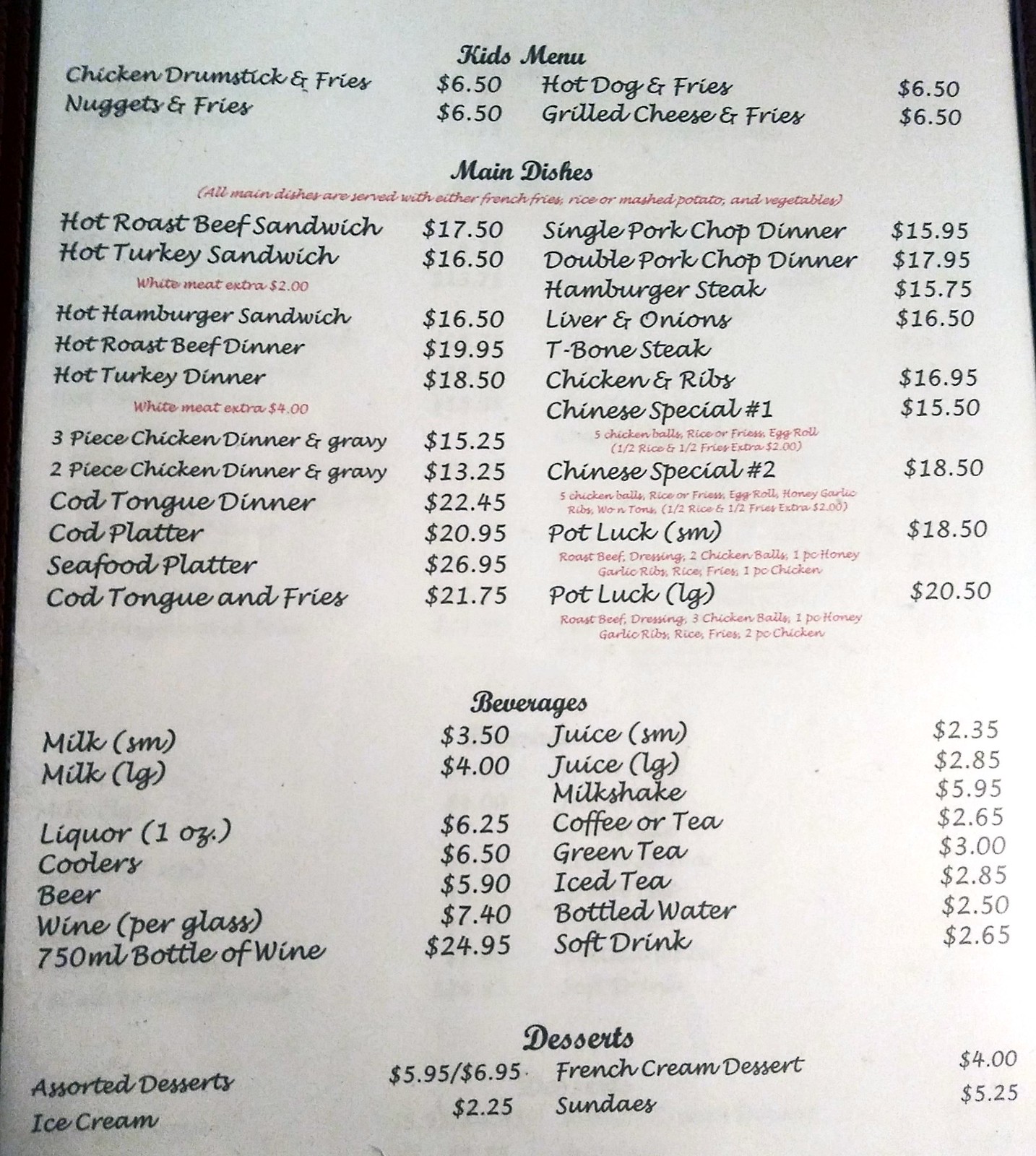The image captures a restaurant menu presented against a very white background. At the top, in bold text, the words "Kids Menu" are prominently displayed. Below this heading, the menu lists three kid-friendly meal options: 

- Chicken Drumstick and Fries - $6.50 (left side)
- Hot Dog and Fries - $6.50 (right side)
- Nuggets and Fries - $6.50 (left side)
- Grilled Cheese and Fries - $6.50 (right side)

All items on the Kids Menu are priced at $6.50.

Underneath the Kids Menu section, the "Main Dishes" section is also presented in bold text. Accompanying the main dishes heading, there is a line in red text indicating that all main dishes are served with a choice of french fries, rice, or mashed potatoes, and vegetables. The main dish options are divided into two columns:

Left side:
- Hot Roast Beef Sandwich - $17.50
- Hot Turkey Sandwich - $16.50 (with an additional $2 for white meat, noted in red text)

Right side:
- Single Pork Chop Dinner - $15.95
- Double Pork Chop Dinner - $17.95

The menu continues with approximately eight more entrées listed in similar fashion on both the left and right sides.

Further down the page, there is a "Beverages" section in bold text, located near the center of the menu. This section enumerated seven or eight beverage options on both left and right sides of the menu.

Lastly, a "Dessert" section, also written in bold, is featured with about four dessert options.

Overall, the comprehensive menu is well-organized into distinct sections, each clearly highlighted and structured for easy reading.